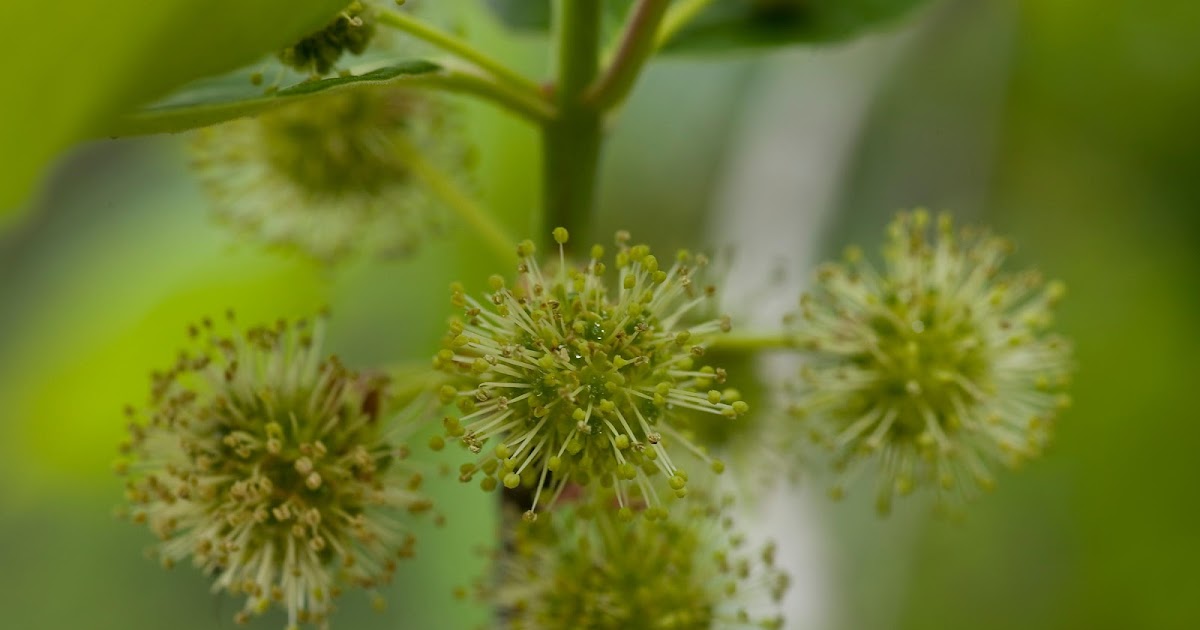This detailed close-up photograph captures a unique plant that resembles a green dandelion. The focal point of the image is the central plant, which features numerous soft, spiky structures ending in tiny bulbs or pods. This unusual plant appears to be in an early blooming stage, as evidenced by the green color and budding bulbs. Surrounding the central plant, there are additional similar plants visible in the background, though they are blurred. The composition highlights the fascinating details of the main plant's stem and spiky bulbs, which seem to be preparing for pollination, possibly aiming to attract bees with their potential nectar and pollen. Above the plant, some leaves can be seen, adding to the intricate natural scene. The image offers a glimpse into a moment of transformation, emphasizing the plant's readiness to spawn and propagate.